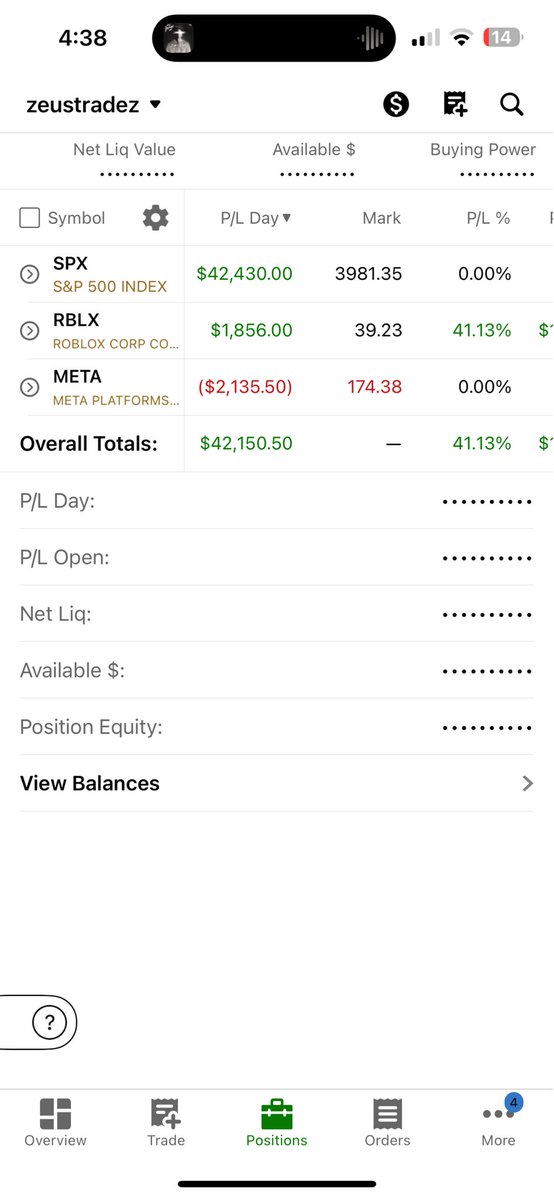This is a detailed screenshot from a mobile stock tracking app displaying the stock prices and performance of various companies. The screen prominently features the S&P 500 index, Roblox Corporation (RBLX), and Meta Platforms Inc. (META). Data is presented in several columns: 'P&L for the current day' shows the profit or loss for each stock, 'Mark' displays the current market price, and 'P&L %' highlights the percentage change in profit or loss. A navigational tab at the bottom allows users to view their balances, suggesting that this app tracks personal investment portfolios. Additional navigation tiles for 'Overview,' 'Trade,' 'Positions,' 'Orders,' and a 'More' button are also visible at the bottom of the screen, providing easy access to various app functionalities.